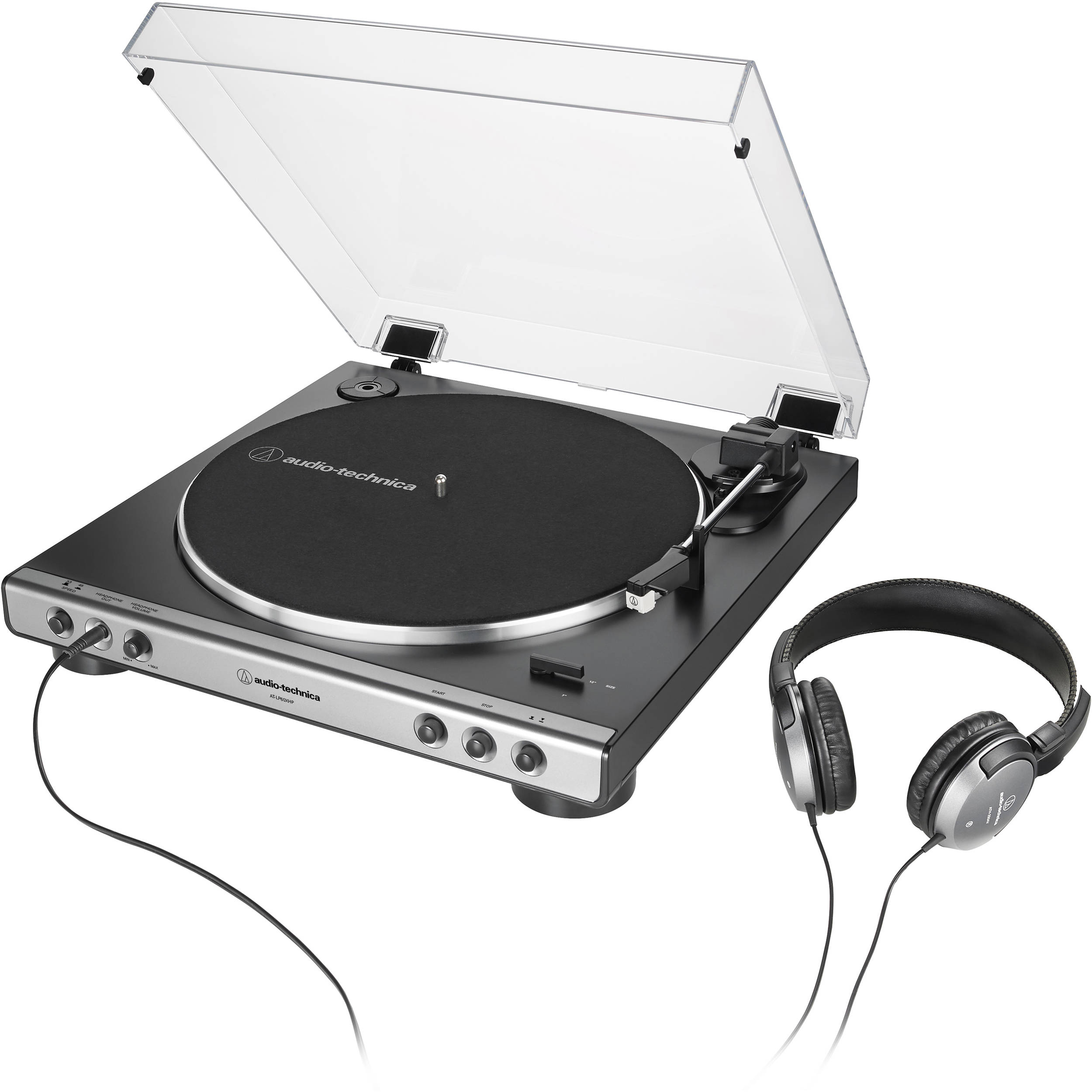This image showcases a modern yet nostalgic Audio-Technica record player, presented on a neutral white background that makes it visually suitable for listings like on eBay. The player, encased in a protective plastic cover, features a monochrome color scheme with sleek black, gray, and chrome elements. The square-shaped turntable prominently displays the Audio-Technica brand name both on the top and front. The setup includes five front-facing knobs and an earphone jack, into which silver and black headphones are plugged, resting to the right of the player. The vinyl player itself is positioned at a slight angle, approximately 30 degrees to the left of the viewer, highlighting its detailed construction, including a centered, opaque black vinyl and the signature needle mechanism poised for play. This piece of audio equipment, likely produced in the last decade, combines high-tech functionality with a classic vinyl experience.